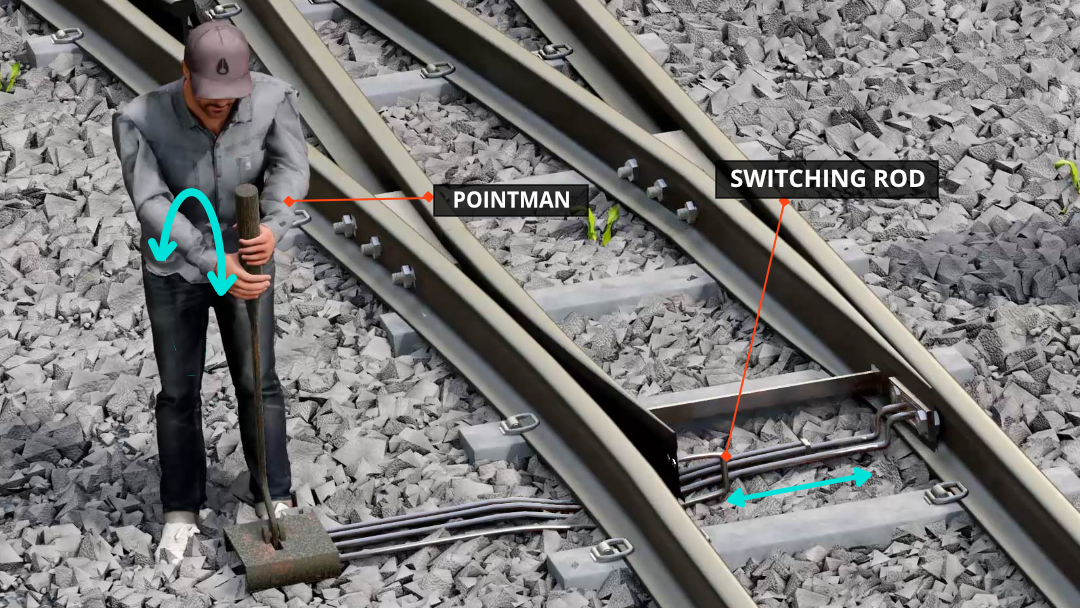The image is a horizontal, computer-generated illustration of a railroad worker, referred to as the "Point Man," standing beside a railroad track where it forks in two different directions. The ground is composed of varied sizes of light gray gravel. The man is dressed in a gray long-sleeved button-down shirt, dark blue jeans, and white sneakers. He wears a cap that could be either a hard hat or a baseball cap. The Point Man is operating a tall metal lever embedded in a concrete base, connected to the railroad tracks via silver pipes.

Two primary elements in the image are highlighted with labels and arrows. A black rectangular box with all-cap white letters, pointed at by an orange arrow, identifies the man as the "POINT MAN." Another orange arrow points to an apparatus on the tracks called the "SWITCHING ROD." Additionally, a blue double-headed arrow is shown between the tracks, indicating some form of motion or connection. The entire scene is set against a backdrop of gravel, including the dark gray railroad tracks that intersect and overlap in the center of the image.